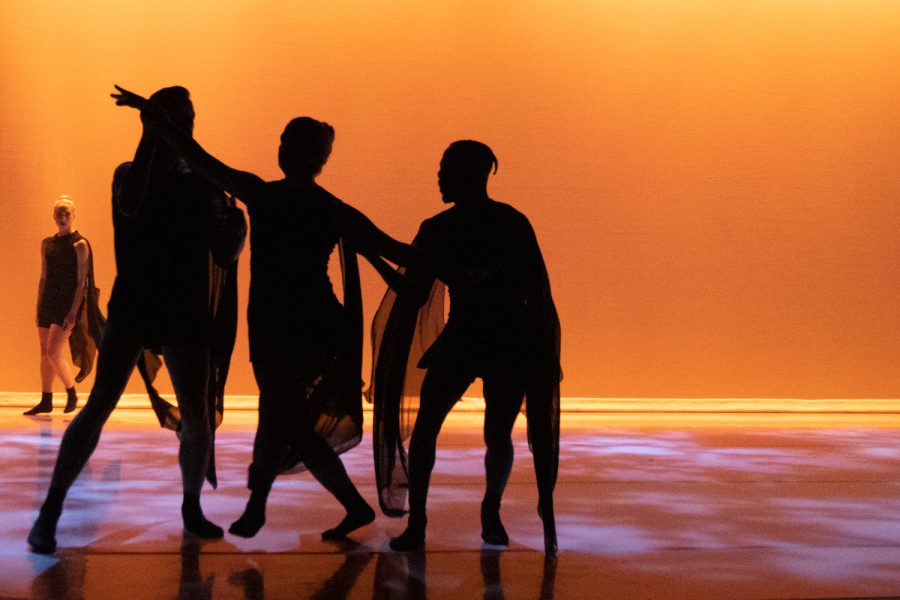The image captures a vibrant performance on a stage with a striking orange and yellow backdrop. The stage flooring features a gradient of pinks and reds, illuminated by a bright yellow baseboard where it meets the wall. The lighting casts the three central dancers into shadowy silhouettes, emphasizing their movements against the colorful background. The central figure appears to be a woman, flanked by two men, all dressed in mesh-like attire. To the far left, a woman in a black dress with blonde hair and black shoes stands slightly in the background, possibly a supporting dancer. The scene's vivid colors and dynamic lighting create a captivating and unique dance performance setting.